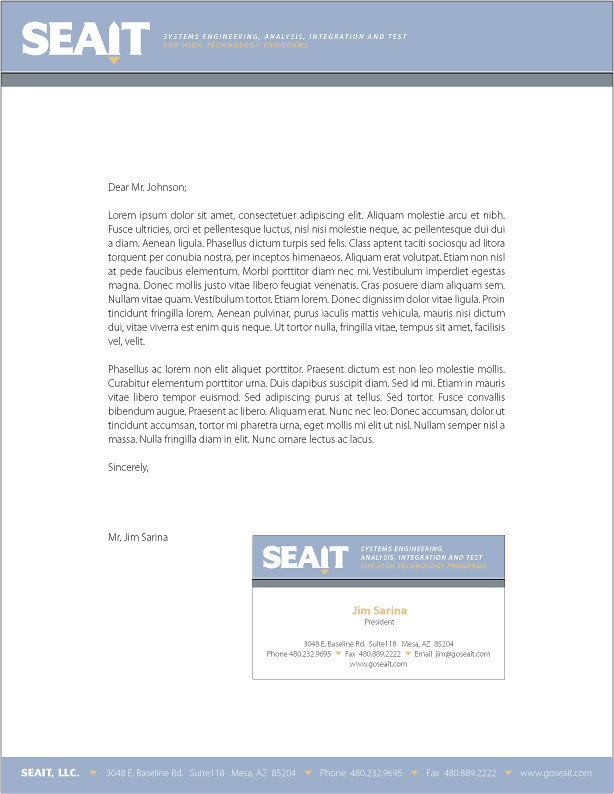The image shows a printout of a professional letter from a company called SEAIT, which stands for Systems Engineering, Analysis, Integration, and Test. The letter is written on white paper with a light bluish-gray border, featuring a sprinkling of yellow font in the name and address areas. The letterhead includes the SEAIT logo prominently, and the text starts in English addressing "Dear Mr. Johnson." Following this English salutation, the majority of the letter is written in an unidentified foreign language. The letter concludes in English with "Sincerely, Miss Jim Sarina." Accompanying the letter is a business card for Jim Sarina, who is identified as the president of SEAIT. The card includes an English-written address, email, fax, and phone number. The overall appearance and design emphasize the professional and corporate nature of the communication.